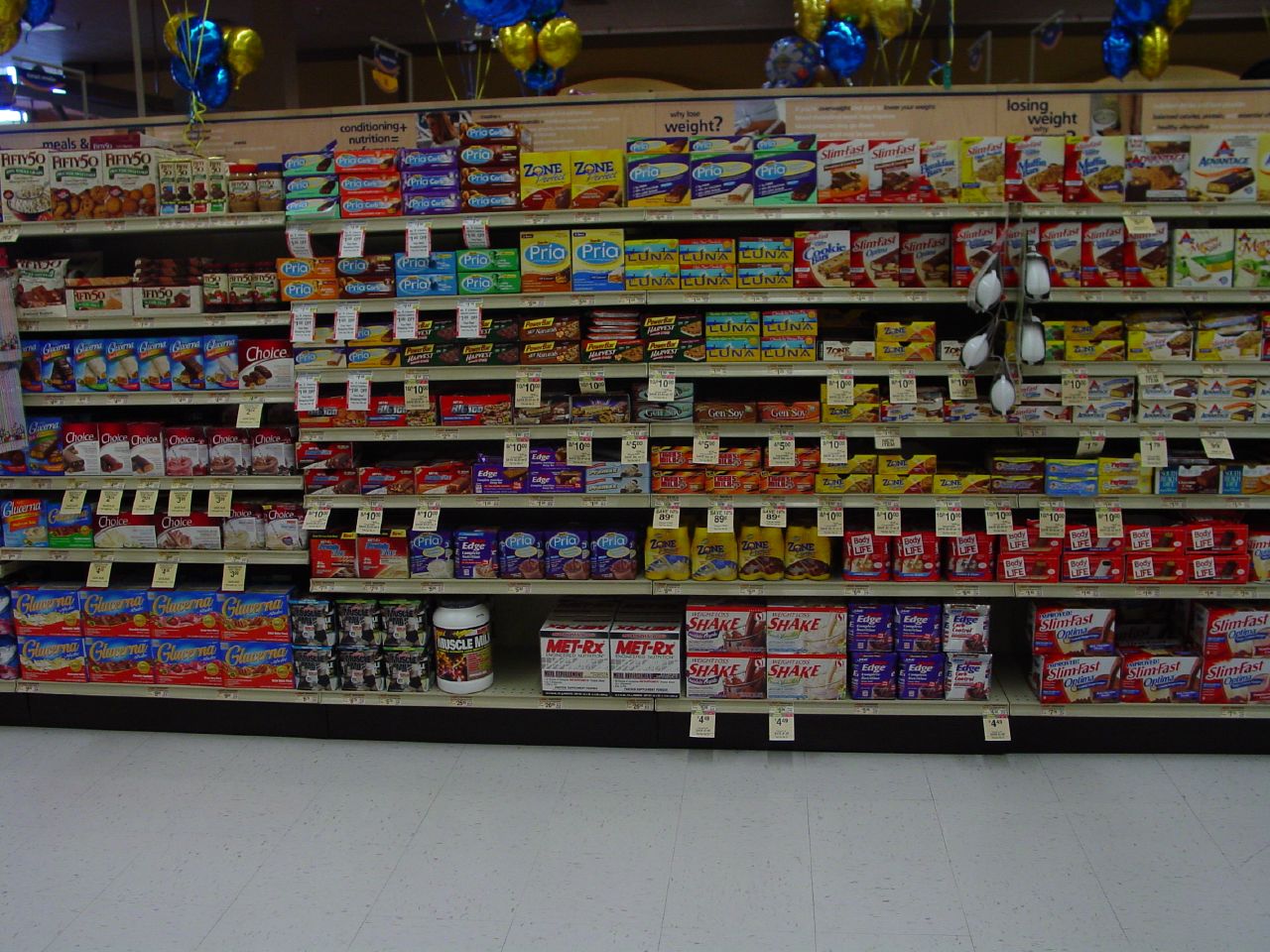This photograph portrays a detailed view inside the breakfast and protein bar aisle of a grocery store, most likely an Albertsons or perhaps a CVS, given the layout and style of the price tags. The image is captured from a first-person POV, facing the shelves directly. The aisle is adorned with festive yellow, blue, purple, and gold balloons at the top, suggesting some sort of celebration or special event. The store's floor is covered in white tiles.

The shelves are stocked with a variety of protein bars, meal replacement shakes, and breakfast options. Prominent products include "Muscle Milk," "Shake," "Slim Fast," "Luna," and "Prio" bars. The products come in various shapes and colors, including red, blue, yellow, orange, and green packaging. 

On the bottom shelves, there are white boxes prominently displaying "SHAKE" in large red letters, alongside "Slim Fast" in red, suggesting meal replacement or protein shakes. The middle shelves feature "LUNA" bars in yellow boxes and various other protein and snack bars. The assortment displayed caters to on-the-go meal solutions with a strong emphasis on health and nutrition. 

Overall, the image effectively captures the diversity and organization of snack options available in this festive and well-stocked grocery aisle.